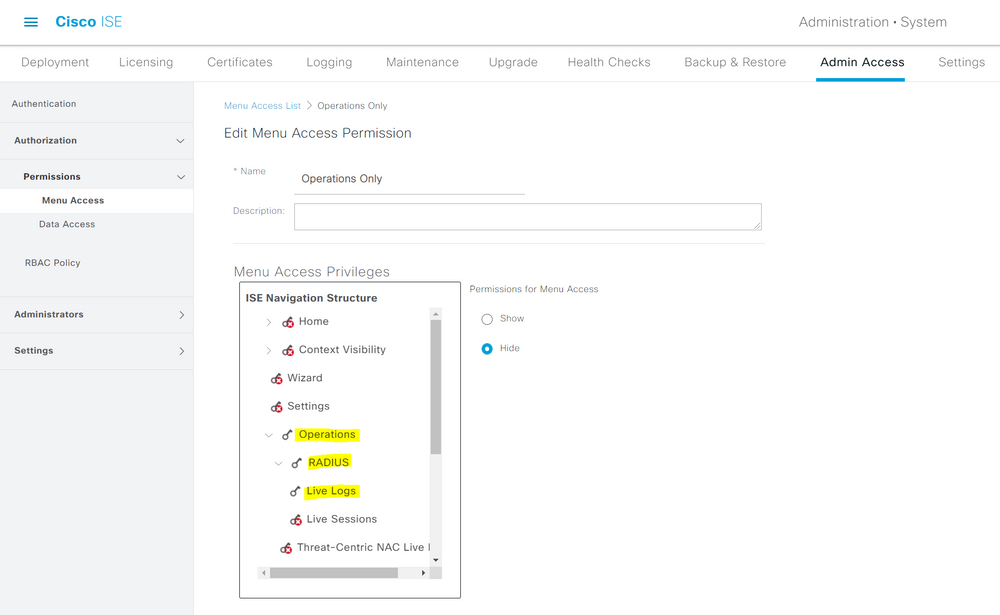This screenshot depicts a system administration interface, likely from Cisco Identity Services Engine (ISE) software, viewed on an unfamiliar laptop or computer. The top left corner features an icon with three horizontally stacked blue lines on a white background, followed by the text "Cisco ISE." In the upper right corner, it reads "Administration > System."

Below this, there is a vertical menu on a gray background with options written in light gray, including:

1. Deployment
2. Licensing
3. Certificates
4. Logging
5. Maintenance
6. Upgrade
7. Health Checks
8. Backup and Restore

The "Admin Access" option is highlighted in black with a blue underline, indicating it is currently selected. Adjacent to this is the "Settings" option.

In the main content area under "Admin Access," there is a section labeled "Menu Access List" with predefined roles and permissions. The role "Operations Only" is displayed, with a text field for "Name" populated with "Operations Only." The "Description" field is empty. 

Beneath this, a section titled "Menu Access Privileges" contains a box listing items such as "ISE Navigation Structure," "Home," "Context Visibility," "Wizard," "Settings," "Operations," "Radius Live Logs," "Live Sessions," "Threat-Centric NIC," and more, though the complete list is cut off. To the right of this box, there is a selection area for "Permissions for Menu Access" with options to show or hide; the "Show" option is currently selected in blue.

On the far left, a toolbar lists additional options including:

1. Authentication
2. Authorization
3. Permissions
4. Menu Access
5. Data Access
6. RBAC Policy
7. Administrators
8. Settings